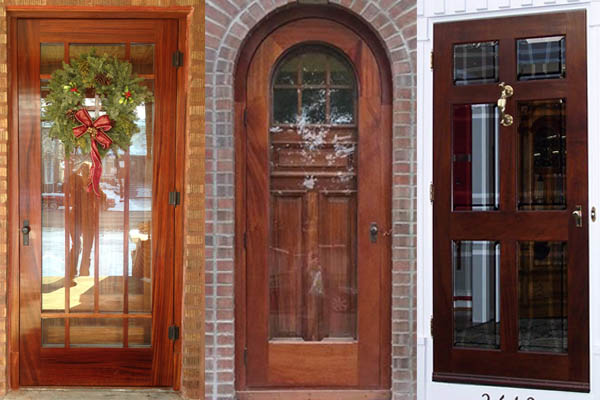This collage showcases three distinct and attractive doorways, each featuring unique styles and shades of brown. The first door on the left is a cedar brown wooden door, predominantly made of glass, accented with three dark hinges and a matching doorknob fixture. It stands against beige brickwork and boasts a festive Christmas wreath adorned with a bow. The second, at the center, is an arched medium brown door framed by red brickwork. This impressive entrance has an outer glass door and an inner wooden door with window panes. The third door on the right is a rich mahogany color, resembling a traditional doorway with a white background. It features six glass panes and an ornate gold knocker. Subtle lettering or numbering under this door hints at a possible catalog reference. Together, these images capture the elegance and diversity in residential entrance designs.